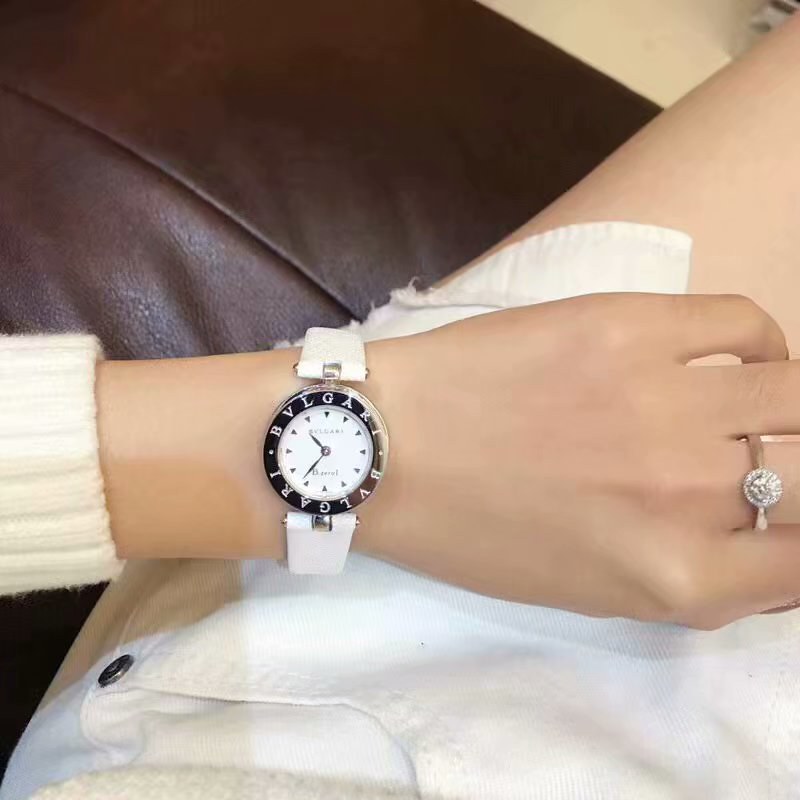In this photograph, the focal point is a woman's arm and wrist extending from the left to the right side of the image. Her hand, of a light skin tone, shows off a white-banded wristwatch by Bulgari, displaying a minimalist design with a white face, black trim inscribed with "B-V-L-G-A-R-I," and no numerals, set to approximately 10:36. The woman is wearing an ivory sweater with the cuff visible on her wrist. Her fingers, cut off at the knuckles by the edge of the photo, feature a striking diamond ring with a yellow band on the middle finger.

The background offers additional context, suggesting the angle is from the woman's perspective, looking down onto her lap and an upholstered chair. In the top left corner, part of a dark burgundy or brown leather-looking seat is visible. Her leg stretches diagonally from the bottom left to the top right, with her waist clad in a white skirt or shorts, leading to a bare thigh that is visible down to just above the knee. The intricate details of her hand, wristwatch, and the subtle background elements create a rich, layered scene.